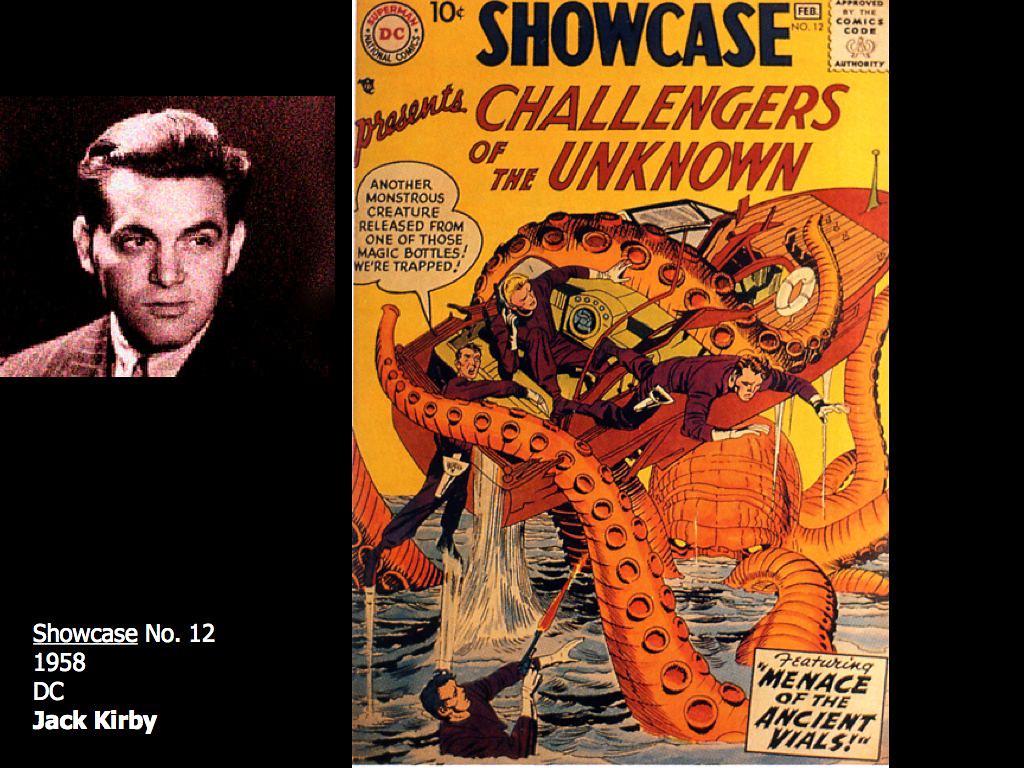This image features a black background with two primary elements. On the left side, there is a black-and-gray portrait of a white man with his hair combed back, dressed in a suit. Below this portrait, white text reads "Showcase No. 12, 1958, DC, Jack Kirby," suggesting that the man depicted is Jack Kirby. To the right, the image showcases an old DC comic book cover titled "Showcase Presents Challengers of the Unknown." The comic book cover, predominantly yellow, illustrates a dramatic scene where a colossal octopus, or Kraken, is attacking a boat, causing people to fall into the water. One man in the water is shooting at the creature, while another man on the boat exclaims, "Another monstrous creature released from one of those magic bottles! We're trapped!" The comic book is also labeled with text in the upper left corner that reads "Superman, DC National Comics" and text in the bottom right corner that states "Featuring Menace of the Ancient Vials." The comic book is slightly off-center with a larger black border on its left side where Jack Kirby's portrait is placed.